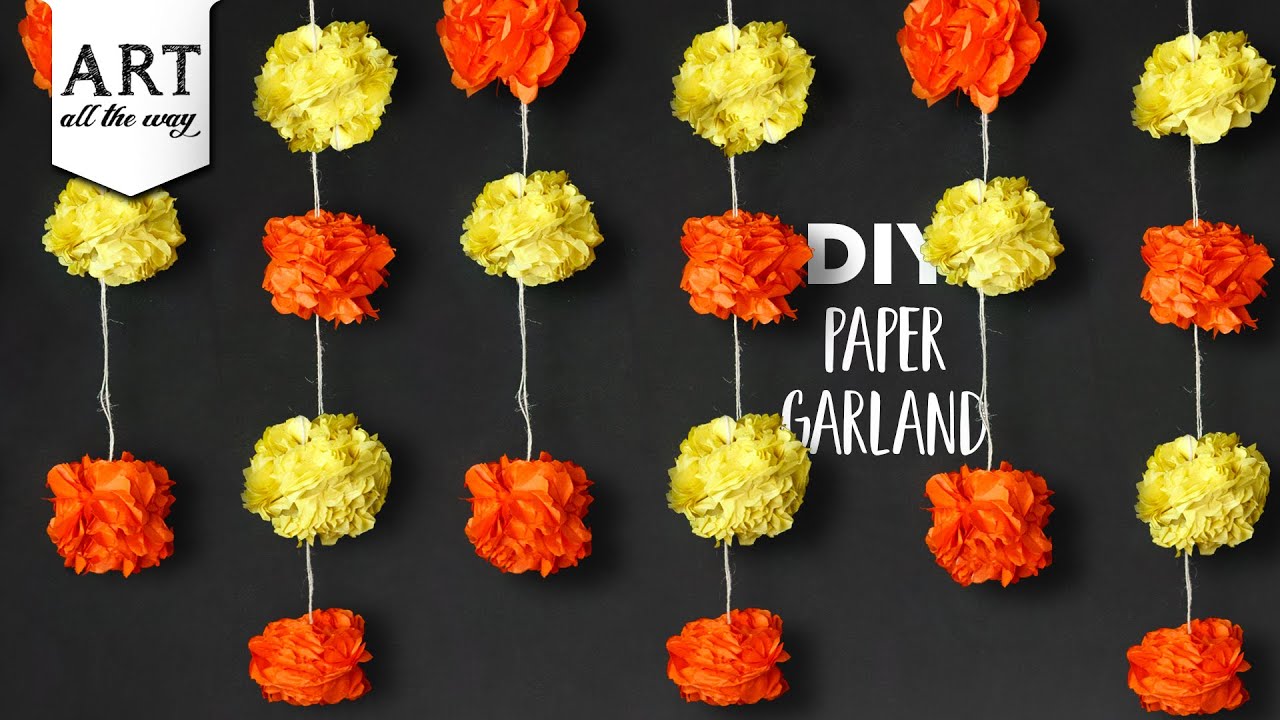The image captures a vibrant DIY art project featuring six vertical strings, each adorned with alternating yellow and orange fluffy tissue paper balls, creating a visually engaging pattern that alternates its hues in a staggered yellow-orange sequence. These white strings hang down from the top of the photograph, extending to the bottom against a predominantly gray background, which resembles a chalkboard with a slight texture suggesting a wall. In the upper left corner, a small white flag with a shield shape proudly displays the text "Art All the Way" in bold black font. To the right, partially hidden behind some of the colorful paper balls, the words "DIY Paper Garland" are written in a white font, further emphasizing the craft's playful and artistic nature. The arrangement and use of color evoke memories of childhood craft projects, imbuing the piece with a sense of nostalgia and creativity.